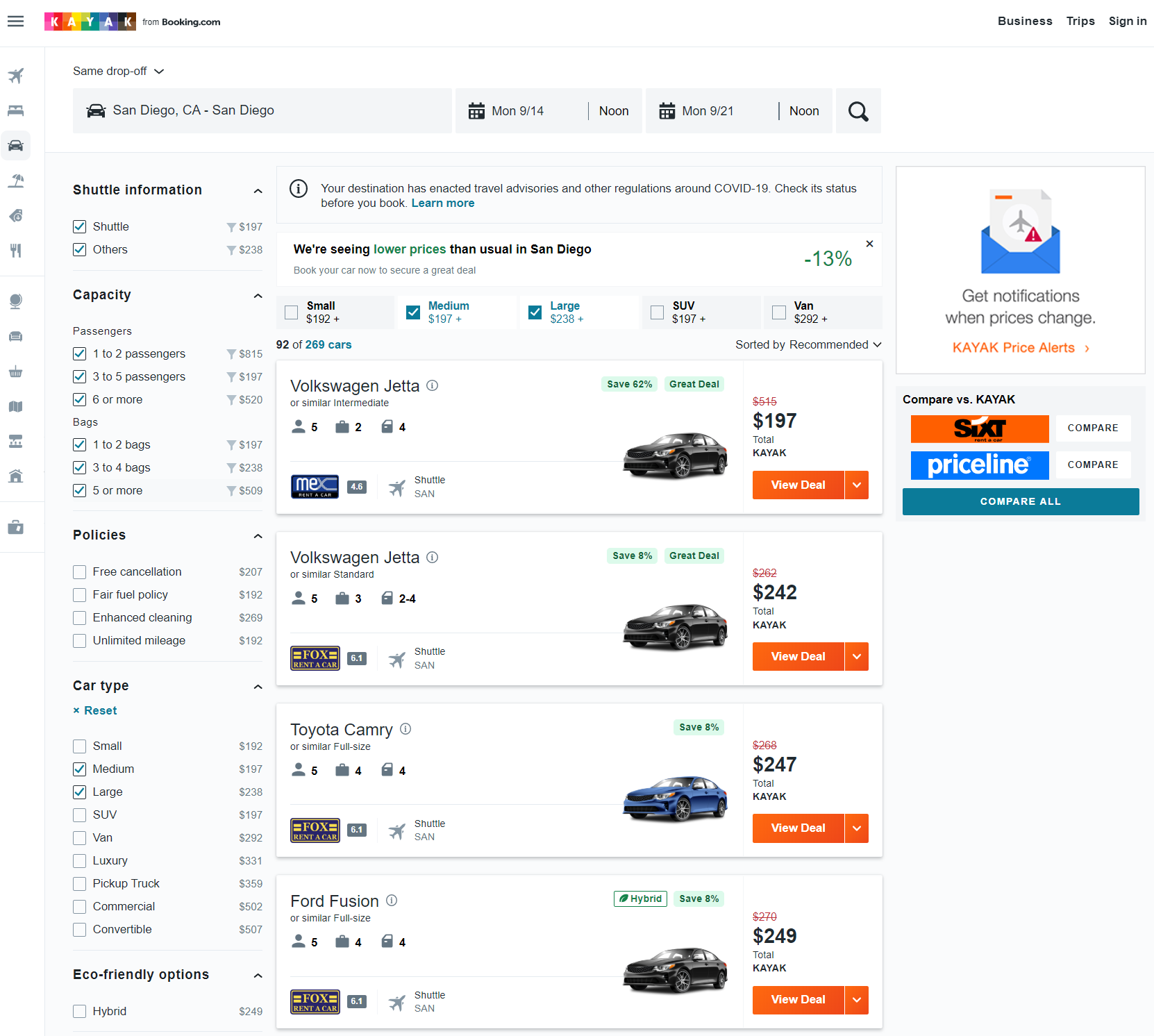**Descriptive Caption:**

The image depicts a web page from a car rental company accessed through the Kayak platform, recognizable by its colorful logo in the upper left-hand corner, accompanied by the "from booking.com" label. The page showcases several filter options allowing users to customize their car rental experience based on criteria such as passenger capacity, luggage capacity, and car type (e.g., small, medium, large, SUV, van, hybrid). The user has selected a rental period starting on Monday, September 14th at noon, with a return on Monday, September 21st at noon, both in San Diego.

The central part of the image features a list of available cars that meet the specified criteria for the selected dates, including their weekly rental rates. The available options highlighted are:

- Volkswagen Jetta for $197 per week
- Volkswagen Jetta for $242 per week
- Toyota Camry for $247 per week
- Ford Fusion for $249 per week

This comprehensive view allows potential renters to easily compare vehicle options and rates to make an informed decision.